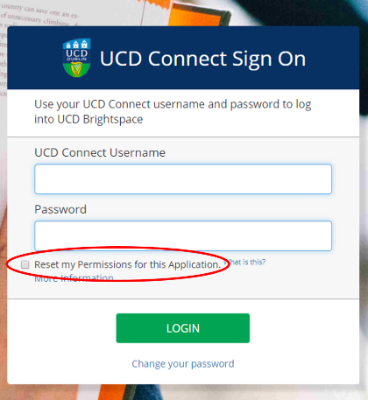The image depicts a web page or application interface displayed on a tablet, featuring a predominately orange background with blue and white accents. Central to the image is a pop-up box with a blue background overlaying the orange backdrop, creating a striking contrast. 

At the top of the pop-up box, there is a crest-like logo adorned with a yellow harp and a series of white lock boxes, signifying it belongs to UCD (University College Dublin). The text on the pop-up reads, "UCD Connect Login or Sign In," followed by instructions: "Use your UCD Connect username and password to log into UCD Brightspace."

Beneath the instructions, there are two input fields: one labeled "UCD Connect Username," and the other labeled "Password." These fields are represented as long, rectangular white boxes with blue outlines. 

At the bottom of the pop-up, there is a hyperlink stating, "Reset my permissions for this application,” which is notably encircled by a red line, indicating emphasis or special attention. The overall layout and details provide a clear and user-friendly interface for logging into the UCD Brightspace system.